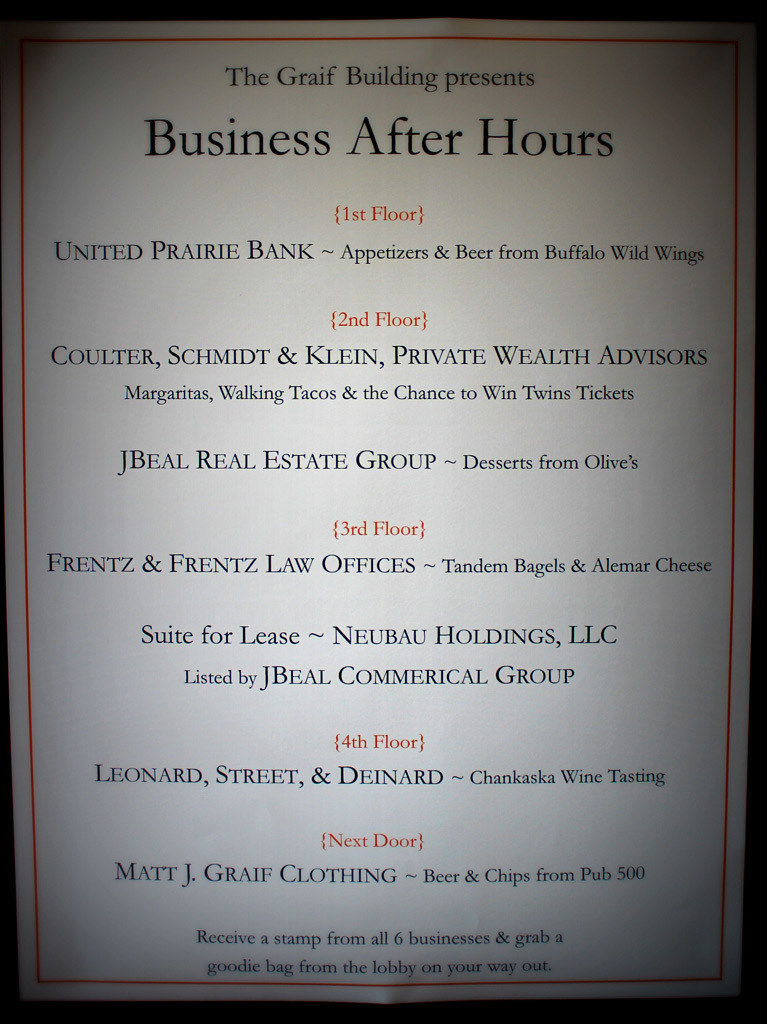The image depicts a detailed sign or flyer for the Graif Building's "Business After Hours" event, set against a white background with a thin orange border, contrasting against what appears to be a black backdrop. The sign, mostly in black and orange text, lists the businesses and activities on each of its four floors. On the first floor, United Prairie Bank offers appetizers and beer from Buffalo Wild Wings. The second floor features Kolder, Schmidt & Kline, Private Wealth Advisors, serving margaritas and walking tacos, with a chance to win Twins tickets, and J. Beal Real Estate Group providing desserts from Olives. The third floor includes listings for Friends and Friends Law Offices, Tandem Bagels and Alamar Cheese, Sweet Frelis, and Nebu Holdings, LLC, managed by J. Beal Commercial Group. The fourth floor houses Leonard Street & Dynard along with wine tasting from Chankaska Creek Ranch & Winery. Additionally, next door features Matt J. Grafe Clothing and beer chips from Pub 500. Attendees are encouraged to receive a stamp from all six businesses and grab a goodie bag from the lobby on their way out.